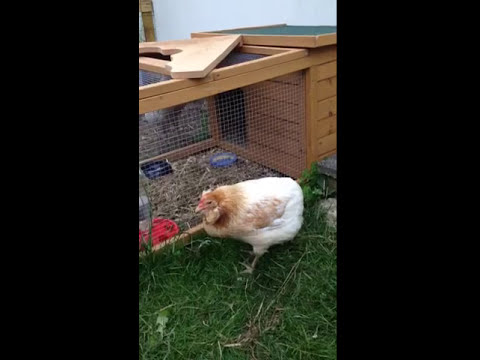In the image, a white chicken with brown feather accents on its head and wings, and a red beak, stands on a patch of green grass, gazing to the left. The setting appears to be a backyard or possibly a small farm. Behind the chicken is a wooden chicken coop, which features meshed wire fencing for containment and a green roof. The coop, with dry grass and straw scattered around, has an interior wooden box for shelter and feeding, containing a red feeding trough and two blue items. There is a prominent detail of a loose wooden slab on top of the coop, raising concern for the chicken's safety. In the foreground, a red wheel is visible, likely a toy for the chicken. The background shows a building with a white wall, adding to the rustic feel of the scene. The image is bordered by thick black bars on each side, framing the picturesque farm-like environment.